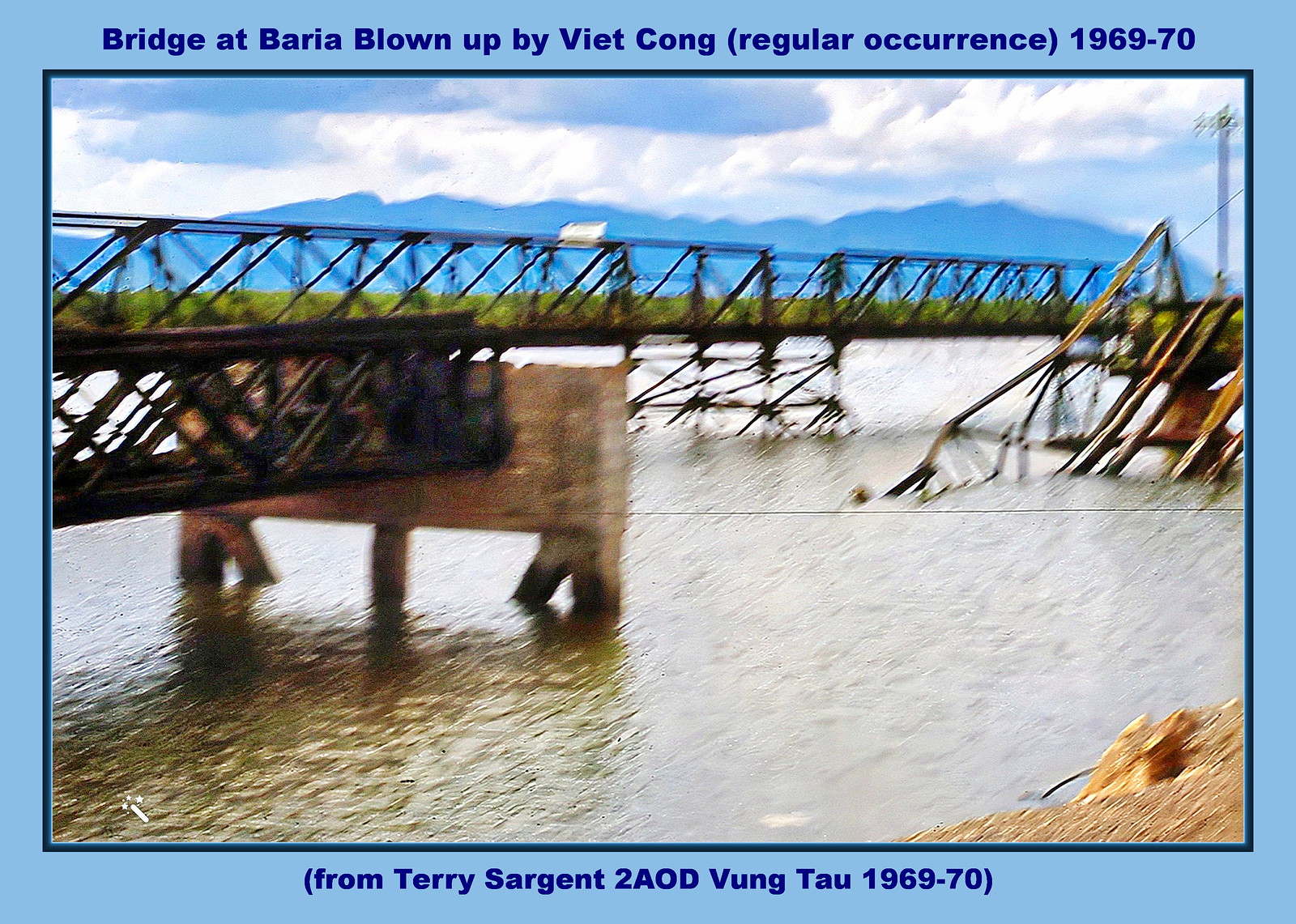The image, likely taken during the Vietnam War, depicts a heavily damaged metal bridge blown up by the Viet Cong. It is surrounded by a light blue border with dark blue text at the top that reads: "Bridge at Baria blown up by Viet Cong. Regular occurrence 1969-70." Below the image, in similar text, it says: "From Terry Sargent to AOD Vung Tau 1969-70." The photo features a blurry and possibly shaky view with a body of greenish-brown water in the foreground and a small portion of the shore visible in the lower right corner. In the background, misty blue hills and a cloudy sky with white and gray clouds can be seen. The central focus is on the bridge, which spans horizontally across the middle of the image. The left section remains intact, while the middle portion is completely missing, having been blown up and partially submerged. The bridge showcases metal trusses and has some parts held up by concrete. In the background, another narrower bridge, possibly a walkway bridge, is visible, also constructed of metal.